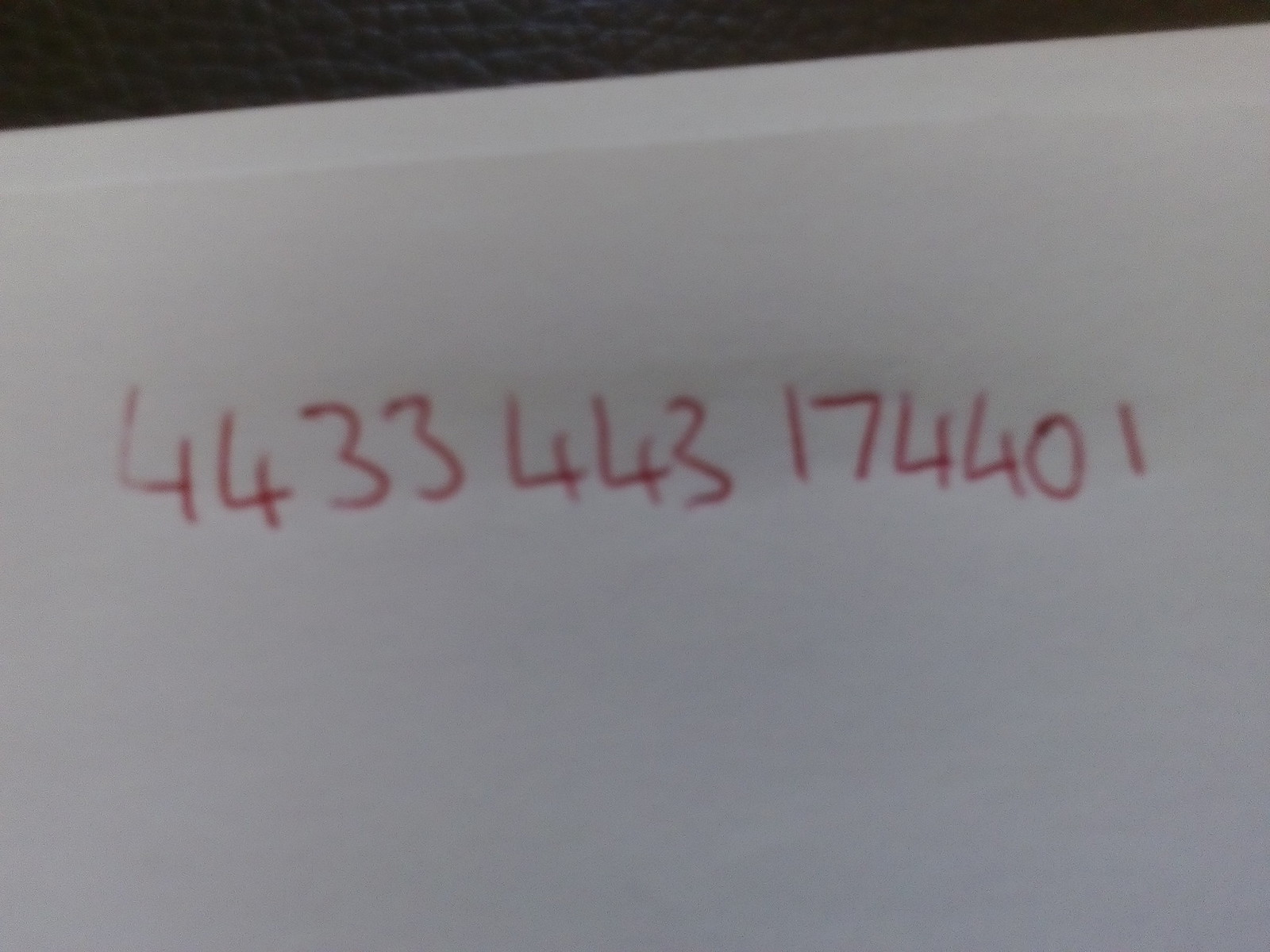This color photograph, slightly wider than it is tall, predominantly features a white sheet of paper occupying almost the entire frame. The paper, which has a faintly darkened tint, leaves a small sliver of a black background visible at the very top, which narrows from right to left. Somewhat uneven at the top edge, the paper appears possibly folded or thicker there, enhancing the impression of depth. Spanning nearly the full width of the paper, a sequence of red ink numbers — "4433443174401" — is inscribed across the center, creating a striking contrast against the predominantly white and subtly shadowed surface.